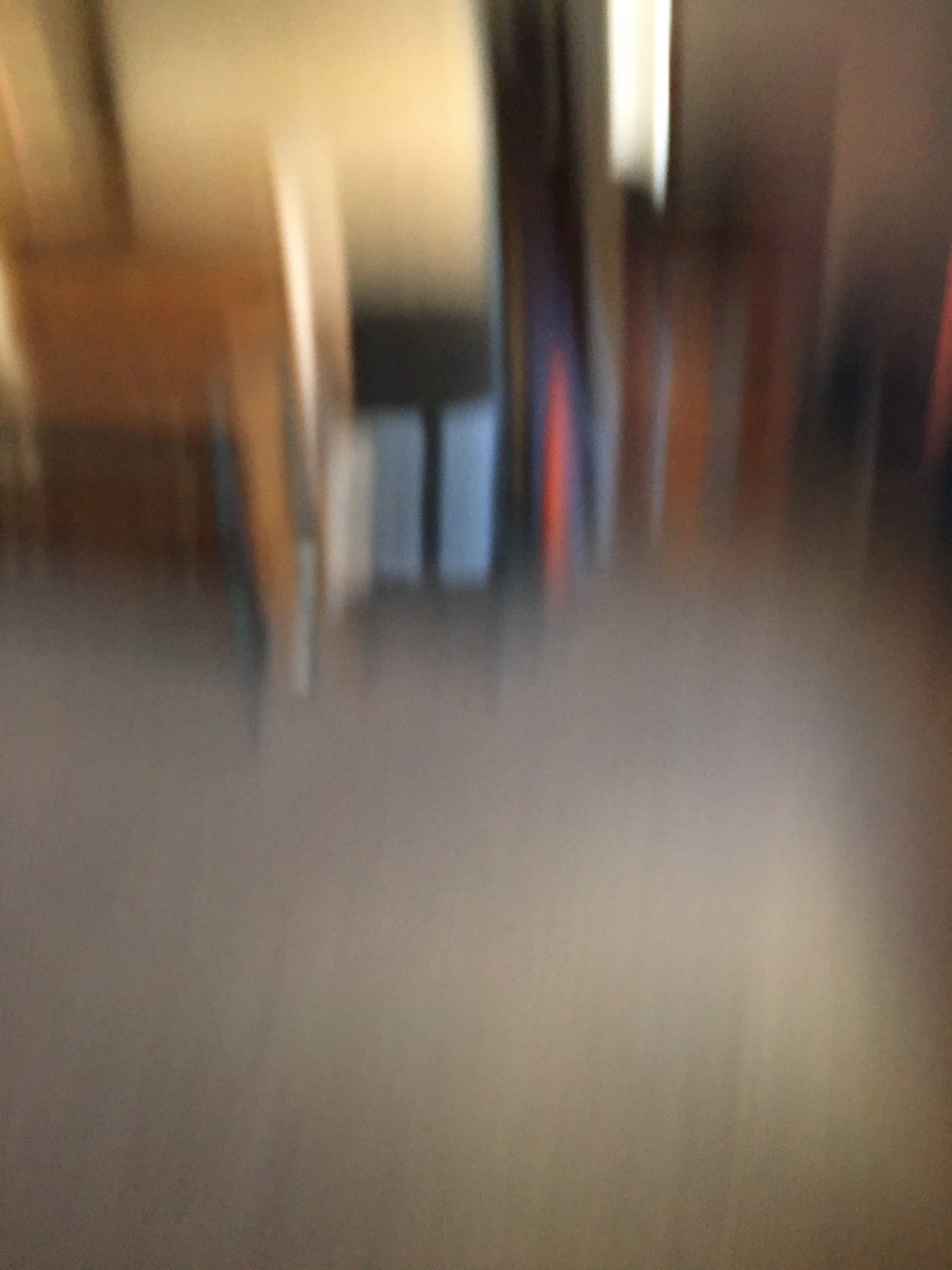The image depicts an indoor room captured in a highly blurry photograph, seemingly taken with a personal camera or cell phone. The room features light tan or beige walls and a floor with a mix of gray and brown hues. Although the blurriness makes it challenging to distinguish specific objects, there appear to be items made of wood and colored elements in red and blue. Vertical streaks suggest that the camera might have been moved during the shot, contributing to the distortion. There's an indication of sunlight filtering through a window, adding patches of light to the scene. Additionally, the photo reveals what might be the opening to another room. The overall composition includes a table and possibly a chair, captured within a rectangular frame, but due to the significant blur, the precise details remain unclear.